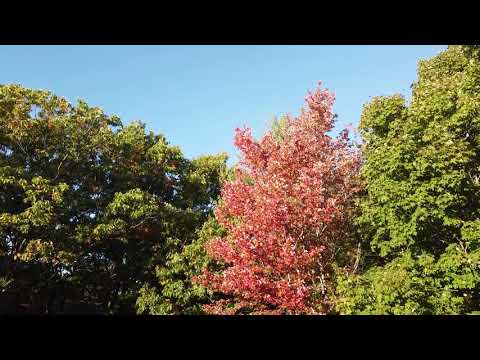The image captures the tops of several tall trees arranged within a square frame, with thick black borders at the top and bottom. In the left section, there are many green trees that appear slightly less vibrant and somewhat sparse, allowing the bright blue sky with a few low clouds to peek through. The middle of the image showcases a very prominent and colorful tree, notable for its rich reddish-pink or coral-colored leaves, suggesting it could be autumn. It stands out against the surrounding foliage, adding a striking contrast. The right side displays another set of lush, green trees, denser and more vibrant than those on the left. These trees, like their counterparts, stretch from the image's bottom to the top, with the clear, cloudless sky providing a serene backdrop.